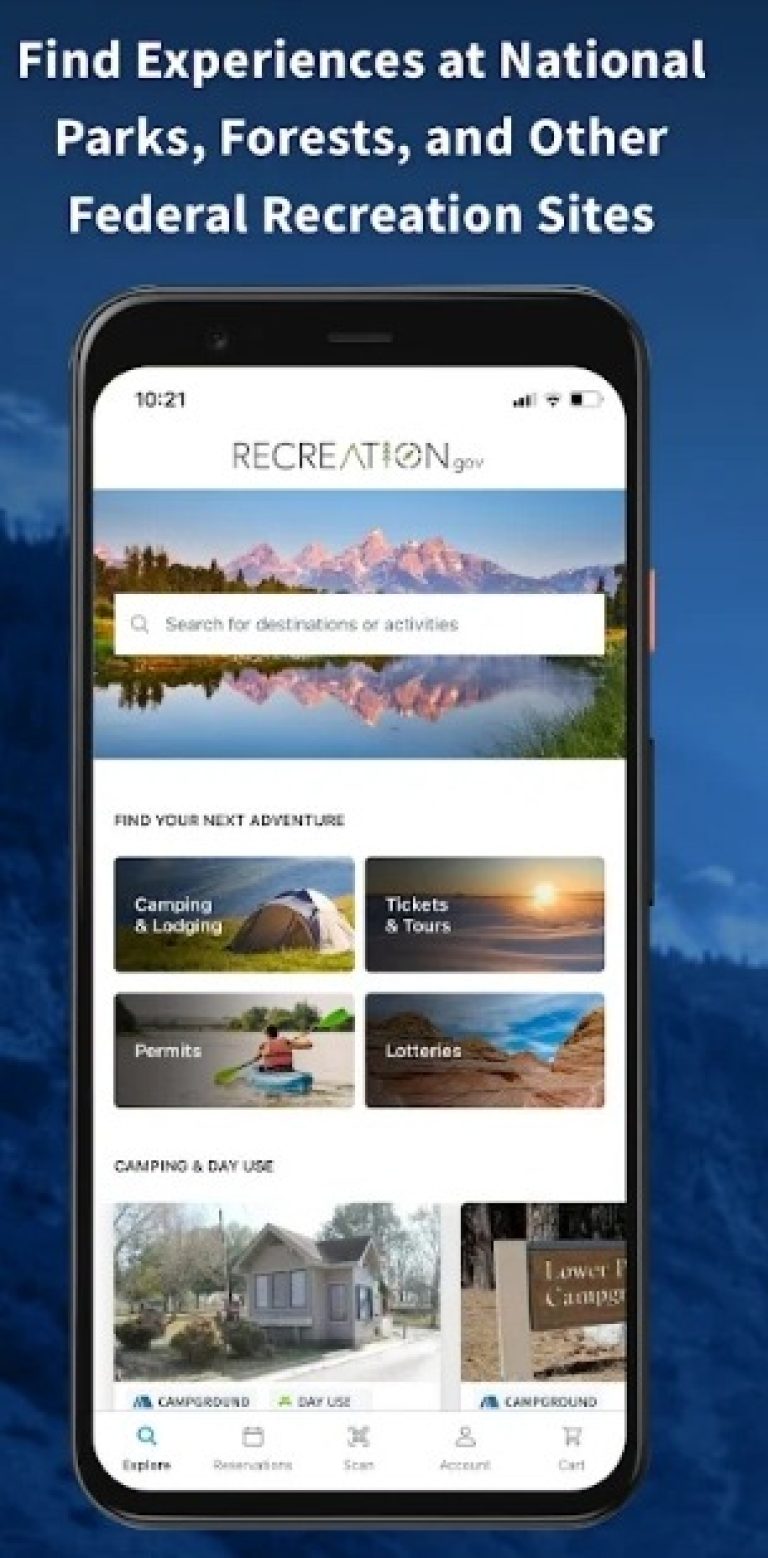This vertical rectangular image features a predominantly blue background, suggesting a serene outdoor environment. The background, tinted with a blue overlay, depicts a sky with clouds visible on the left side and slightly lower than the midpoint on the right side. The horizon and possible ground elements blend harmoniously into this blue landscape.

At the very top of the image, white bold text reads, "Find experiences at national parks, forests, and other federal recreation sites." Below this text, an image of a smartphone occupies the center of the frame. The smartphone's screen displays its black notification bar at the top, showing "10:21" on the left corner, battery status on the right corner, and the term "recreation" in white font at the center, followed by what appears to be ".gov".

The phone screen prominently features a picturesque scene of mountains in the center, tall trees on the left, and grassy terrain leading to a body of water at the bottom. The water surface captures a mirror-like reflection of this idyllic landscape. Overlaying this image is a horizontal white rectangular pop-up with a search icon and the text, "Search for destinations or activities."

Further down on the phone's screen, crisp white text invites users to "Find your next adventure." Below this call to action, four horizontal rectangular boxes display various recreational options:
1. "Camping and something" (illegible) with an image of a tent and outdoor grass.
2. "Tickets and tours" with a striking sunset image.
3. "Permits" accompanied by a picture of a person kayaking on water.
4. "Lotteries" featuring mountains under a blue sky backdrop.

At the bottom of these options, additional text reads "Camping and day use," alongside an image that appears to depict a house and a camping sign. The bottom of the phone screen includes the familiar app icons commonly found on mobile devices.

Overall, the image effectively conveys the accessibility and variety of experiences available through federal recreation sites, integrating both visual and textual elements to entice potential explorers.